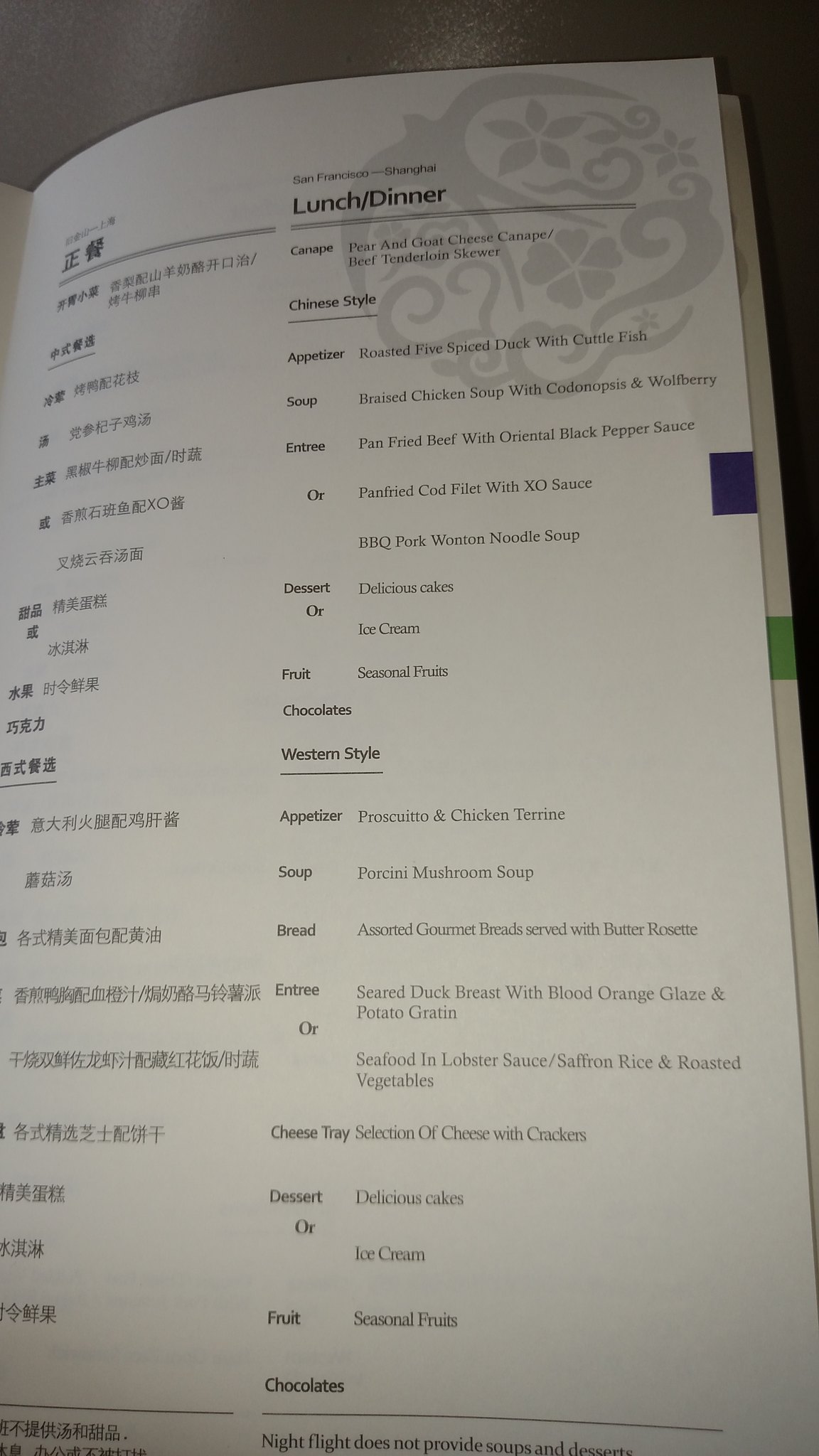The photograph captures a vertically long menu, prominently occupying most of the frame against a dark brown, matte background visible at the very top and slightly on the upper right. In the top right of the menu, a light gray design is visible underneath the text, adding a subtle decorative touch. Towards the middle right of the menu, a small purple rectangle serves as an accent to the paper, while a green rectangle peeks from beneath another page slightly lower.

The left column of the menu features Chinese text, appearing to be neatly arranged in spaced-out rows. Adjacent to this, the right column contains English translations. The menu begins with "San Francisco, Shanghai" at the very top, followed by larger text, "Lunch / Dinner," separated by a long divider. The sections of the menu are meticulously categorized as follows:

**Canape**
- Pear and Goat Cheese Canape
- Beef Tenderloin Skewer

**Chinese Style**
- **Appetizer**
  - Roasted Five Spice Duck with Cuttlefish

- **Soup**
  - Braised Chicken Soup with Codonopsis and Wolfberry

- **Entree**
  - Pan-Fried Beef with Oriental Black Pepper Sauce
  - Pan-Fried Cod Fillet with XO Sauce
  - Barbecue Pork Wonton Soup (not noodle soup)

- **Dessert**
  - Delicious Cakes or Ice Cream
  - Seasonal Fruits
  - Chocolates

**Western Style**
- **Appetizer**
  - Prosciutto and Chicken Terrine

- **Soup**
  - Porcini Mushroom Soup

- **Bread**
  - Assorted Gourmet Bread served with Butter Rosé

- **Entree**
  - Seared Duck Breast with Orange Glaze and Potato Gratin
  - Seafood in Lobster Sauce with Saffron Rice and Roasted Vegetables

- **Cheese**
  - Selection of Cheeses with Crackers

- **Dessert**
  - Delicious Cakes or Ice Cream
  - Seasonal Fruits
  - Chocolates

A note at the bottom mentions that "Night flights do not provide soups and desserts."

The intricate layout and detailed descriptions in both Chinese and English provide a comprehensive overview of the menu offerings, reflecting a blend of Chinese and Western culinary options.